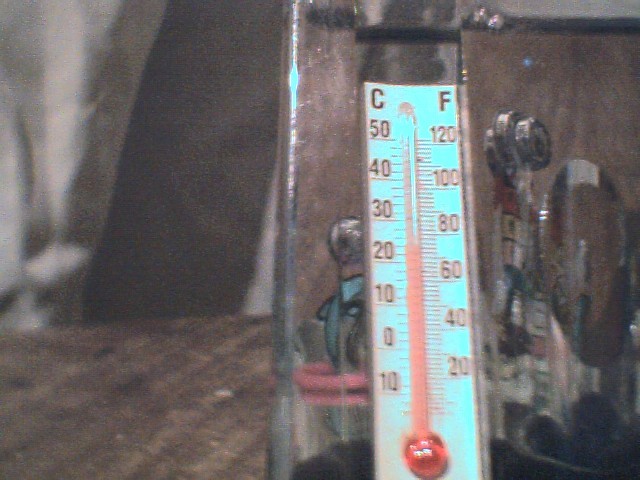The image showcases a classic, tall rectangular thermometer slightly off-center to the right. Encased in a glass jar or cup, the thermometer stands against a white background with a faint light blue tint. The centerpiece of the image is the vivid red liquid, resembling mercury, which indicates a temperature of approximately 70 degrees Fahrenheit. On the top corners of the thermometer, the letters "C" and "F" denote Celsius and Fahrenheit, respectively. The Celsius side shows a descending scale from 50 to -10 degrees, while the Fahrenheit side displays a range from 120 to 20 degrees. Surrounding the thermometer is a subtle floral design painted on the glass covering. This entire setup rests on a brown wooden tabletop. The backdrop consists of dark, tan, grainy-colored long curtains or drapes, adding a textured contrast to the scene.